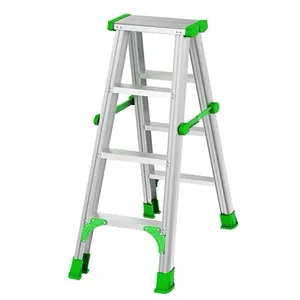The image features a small three-step folding ladder prominently displayed against a pristine, white background. The ladder is constructed from aluminum, showcasing silver rungs and tall rods with visible silver rivets. Bright lime green accents are strategically placed, adding a pop of color to the ladder's design. These green highlights appear as pads around the feet on the forelegs, braces at the bottom of the first step, and on the connecting rods and angles. Additionally, the sides of the top flat area feature green capping, which appears to be made of either plastic or rubber. The ladder is opened up, revealing its structure with three steps on both the front and back sides of the ladder.